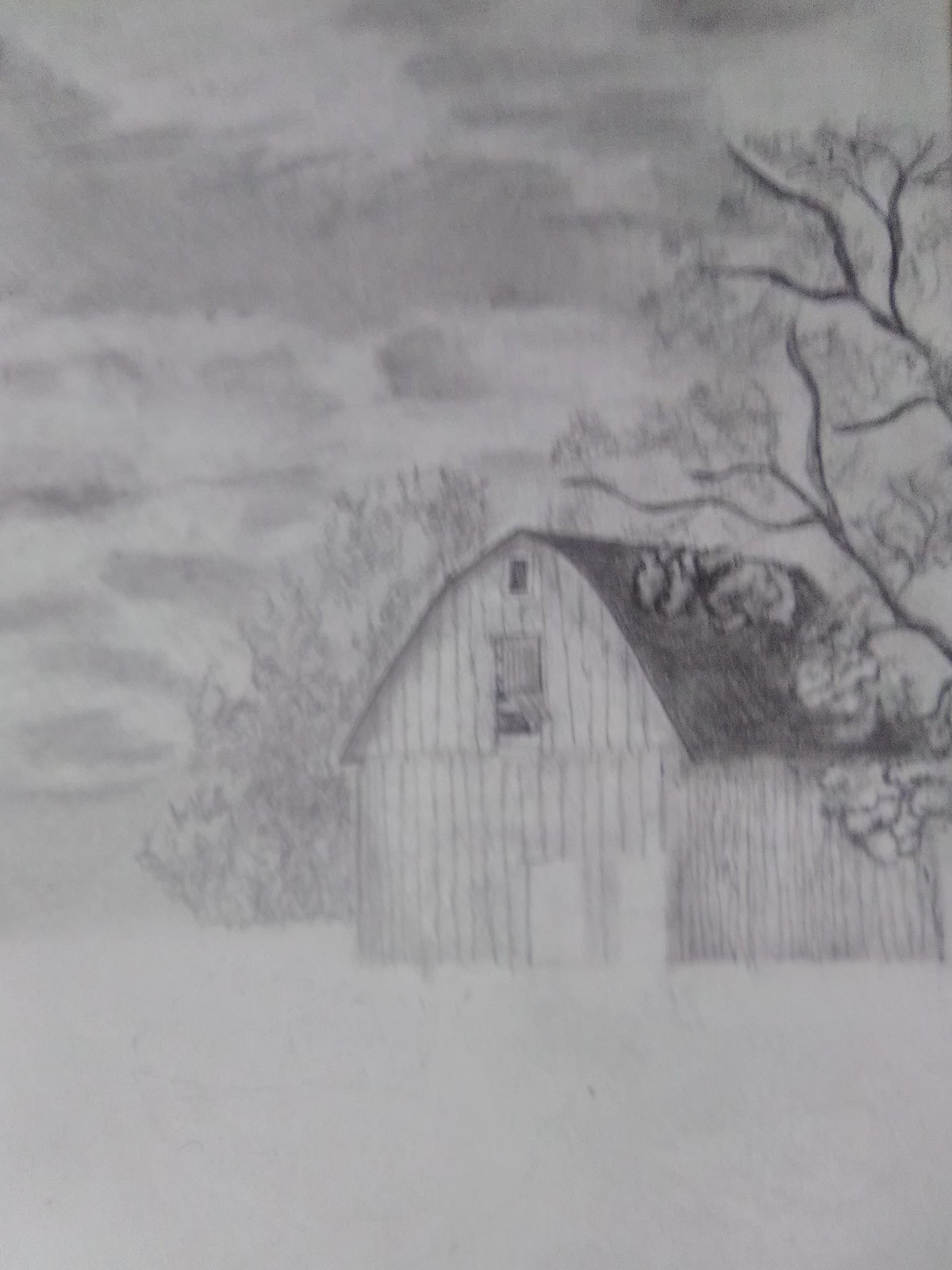This photograph depicts a real-life image of a hand-drawn pencil sketch, captured with a low-resolution camera, resulting in a very blurry and grainy appearance. The sketch itself is primarily done in shades of gray, featuring intricate details on a white sheet of paper. At the center of the image, positioned slightly to the right, is a barn with considerable detail: the lower half showcases numerous vertical lines and an open door leading into a blank white interior. The top half of the barn is marked by a darkly shaded roof with an almost triangular shape, intersected by a horizontal line, and a rectangular window in the middle. Adjacent to the barn, to the right, stand a couple of trees with sparse leaves, their branches extending over the top right part of the image. To the left, behind the barn, is a large bush. The foreground is featureless and white, suggesting either snow or an unfilled area. The sky is heavily shaded, illustrating a stormy or cloudy ambiance with various shades of gray and scattered darker clouds.